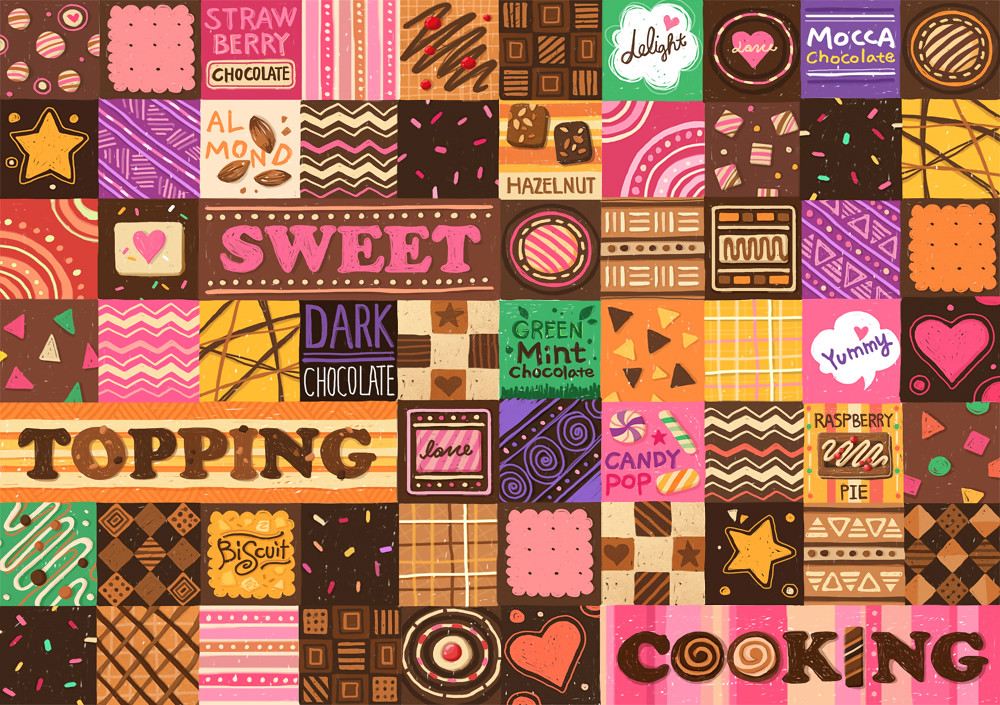The image features a vibrant poster resembling a quilt, filled with around 70 vividly colored squares and rectangles of various shapes and designs. Each section showcases an assortment of colors such as red, purple, brown, green, pink, and tan, all arranged in an intricate, eye-catching pattern. Key sections include a striking brown square with pink writing saying "sweet" in the middle, and a prominent green square labeled "green mint chocolate." Additionally, there's a notable black square with the words "dark chocolate," and a variety of other squares depict delightful food-related themes. Words like "strawberry chocolate," "delight," and "mocha chocolate" are scattered across the poster, enhancing its culinary appeal. Several groupings of squares stand out: one with hazelnuts, another with an adorable red heart, four linked squares with "topping" written on them, and another set in the lower right corner spelling out "cooking." This colorful mosaic of squares not only combines different hues and textures but also fills the entire card with a delightful, candy-themed aesthetic.